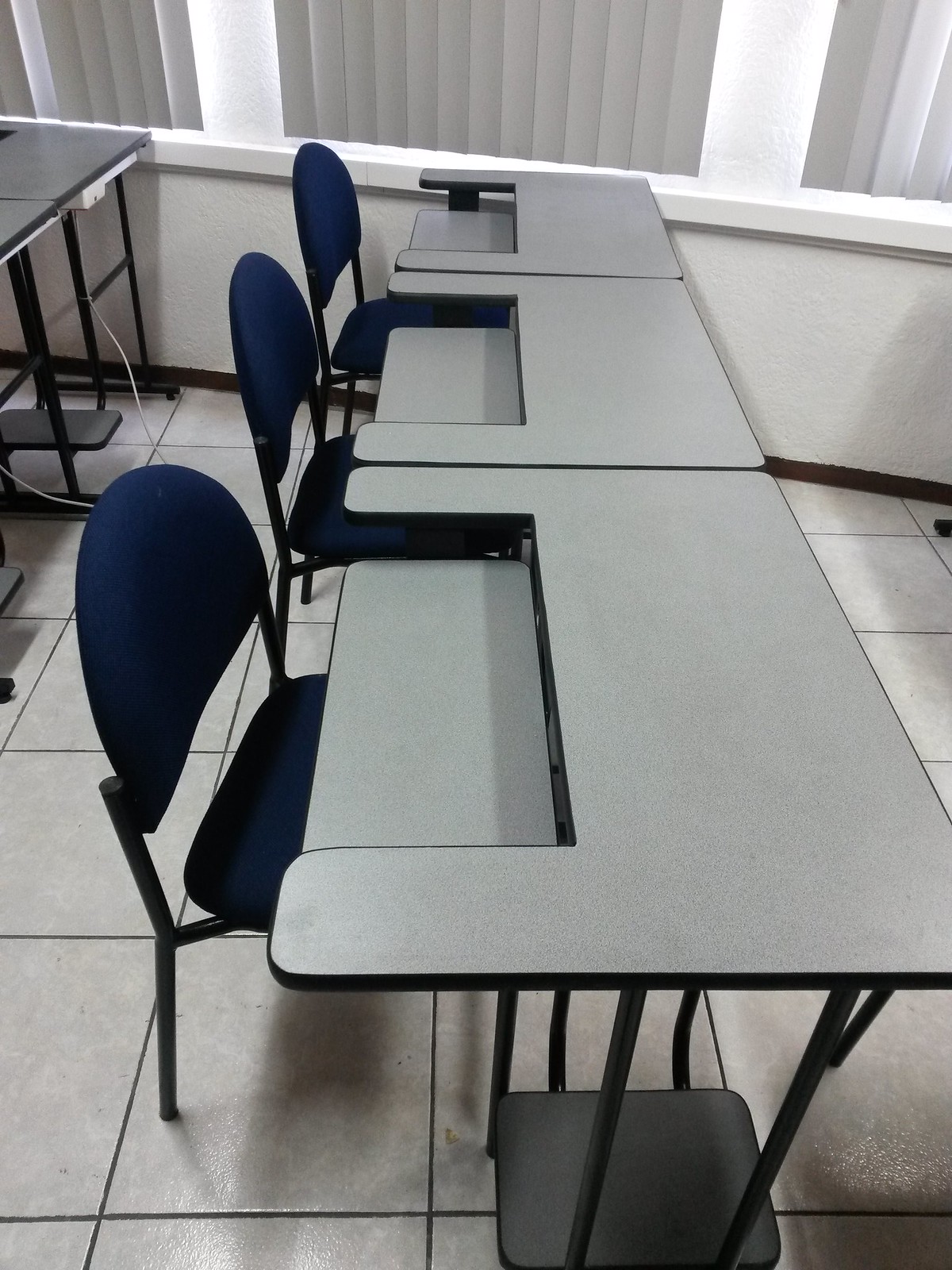This photorealistic image depicts a training center or classroom featuring three gray Formica desks arranged side by side in a neat row. Each desk is a computer-style workstation with a main surface and an inset lower area designed for keyboard use or to accommodate a laptop, ensuring a comfortable typing height. The desks' configuration allows for unobstructed view and access throughout the space. Surrounding the desks are simple, yet sturdy, blue chairs with padded seats and rounded backrests, all supported by a black metal frame. The room's floor is laid with gray tiles, contributing to the functional and clean aesthetic of the space. In the background, white walls host windows adorned with vertical slat blinds, filtering the harsh overhead lighting that casts vague, undefined shadows around the room, enhancing the organized and professional atmosphere.